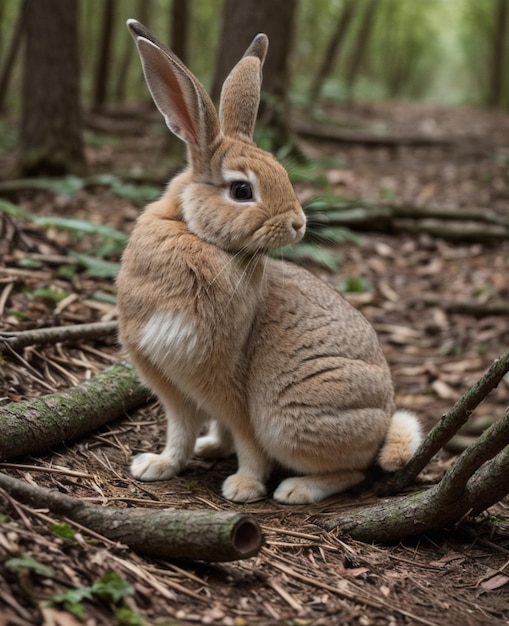This AI-generated image captures a detailed scene of a wild rabbit in a forest setting. The light brown rabbit, adorned with white fur around its eyes, chest, and paws, sits on the ground amid fallen debris and branches, including small twigs and moss-covered wood. The rabbit is positioned in the center of the image, with its front legs directed to the left and its head turned to the right, showcasing its long, upright ears tipped with dark brown or black. Its cottontail is a mix of white and light brown. The backdrop features trees and a forest trail extending into the distance towards the upper right corner, hinting at an overcast day as the scene lacks pronounced shadows, suggesting diffused lighting possibly blocked by the tree canopy. The ground is a mix of brown leaves and natural forest litter, creating an earthy ambiance that encapsulates the rabbit's natural habitat.